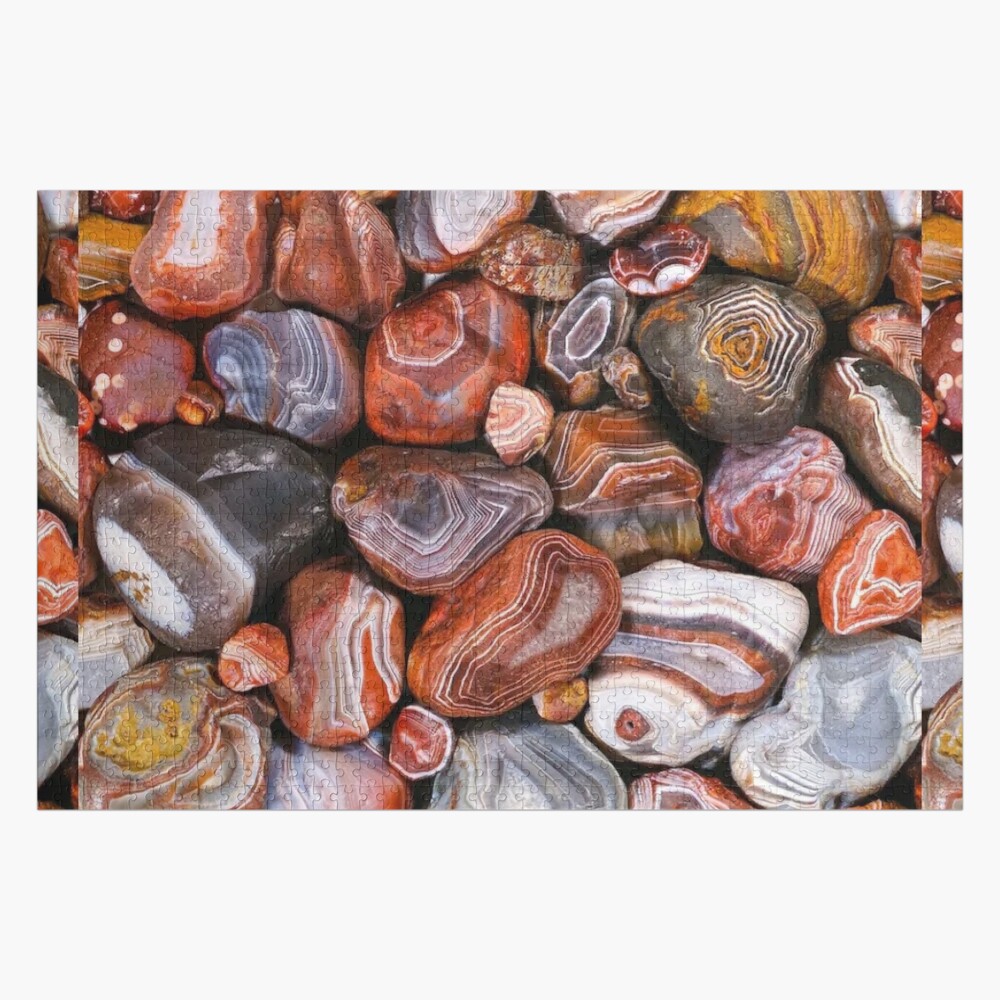The image is a color photograph in landscape orientation, showcasing a diverse and intricately detailed pile of polished rocks. These rocks, closely packed and arranged in a flat layer, display an array of colors including red, brown, black, white, and yellow. Many of these rocks feature elegant, spiral patterns with sections outlined in white, giving them a distinctive and decorative appearance. Some rocks have a smudged look, while others resemble specific shapes or images, such as one appearing to have the face of a dog with a white base, a beige band across where the eyes would be, and a brown spot where the nose might be. The rocks vary in size and have a professionally polished finish, making them appear very shiny and smooth. Surrounding the central pile, the segmented strips of the same photograph are visible, creating a jigsaw puzzle effect in the overall composition. The background of the image is white, further highlighting the vivid colors and intricate patterns of the rocks.